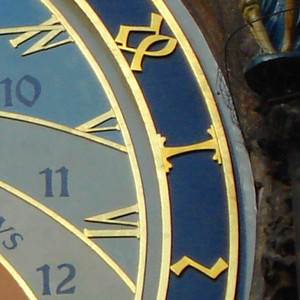This is a close-up photograph of a clock or possibly a measuring device, featuring intricate and detailed elements. The clock face displays the numbers 10, 11, and 12 twice: once in dark blue regular numerals and again in gold Roman numerals. Surrounding the clock are several gold trims and bands, creating multiple concentric circles that enclose the device. The innermost circle has a blue rim, followed by additional gold encasements. The background to the right of the clock is filled with dark shades of brown, blue, and gold, adding to the rich, textured appearance. There are additional details at the bottom left-hand side, including the letter 'S' and possibly other hard-to-make-out letters, contributing to the intricate design.